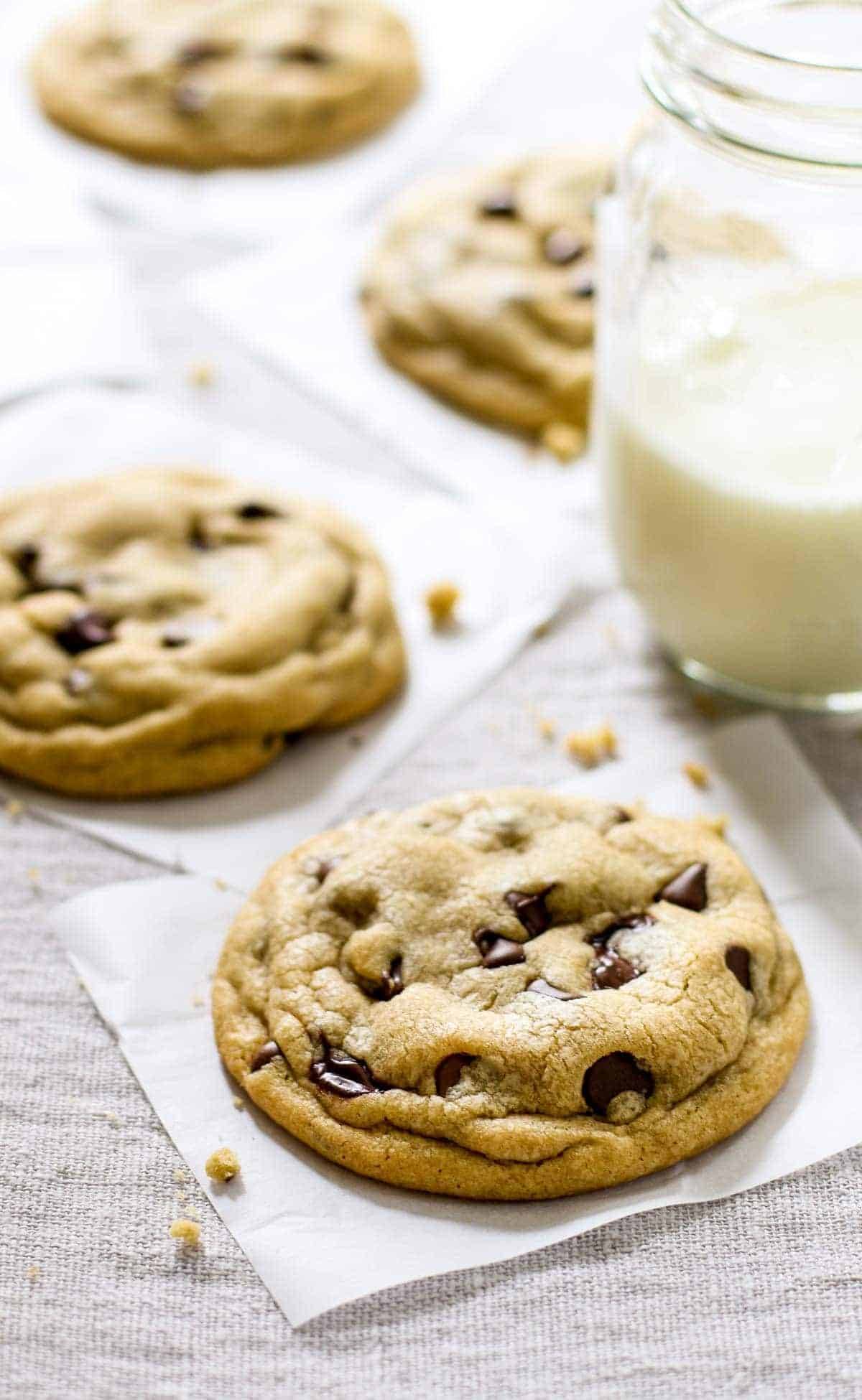The image features four homemade chocolate chip cookies, each resting on individual white squares of parchment paper placed atop a light beige fabric, possibly linen. The cookies are arranged with one in the foreground, one to its left, another partially obscured by a thick mason jar of half-full milk on the right, and the final one blurred in the background. The cookies are generously sized, wider than the jar of milk, with a fluffy texture and a light tan color peppered with melted, dark brown chocolate chips. Crumbs of the cookies are scattered around on the parchment paper and the fabric beneath, emphasizing their crumbly, yet tender consistency.